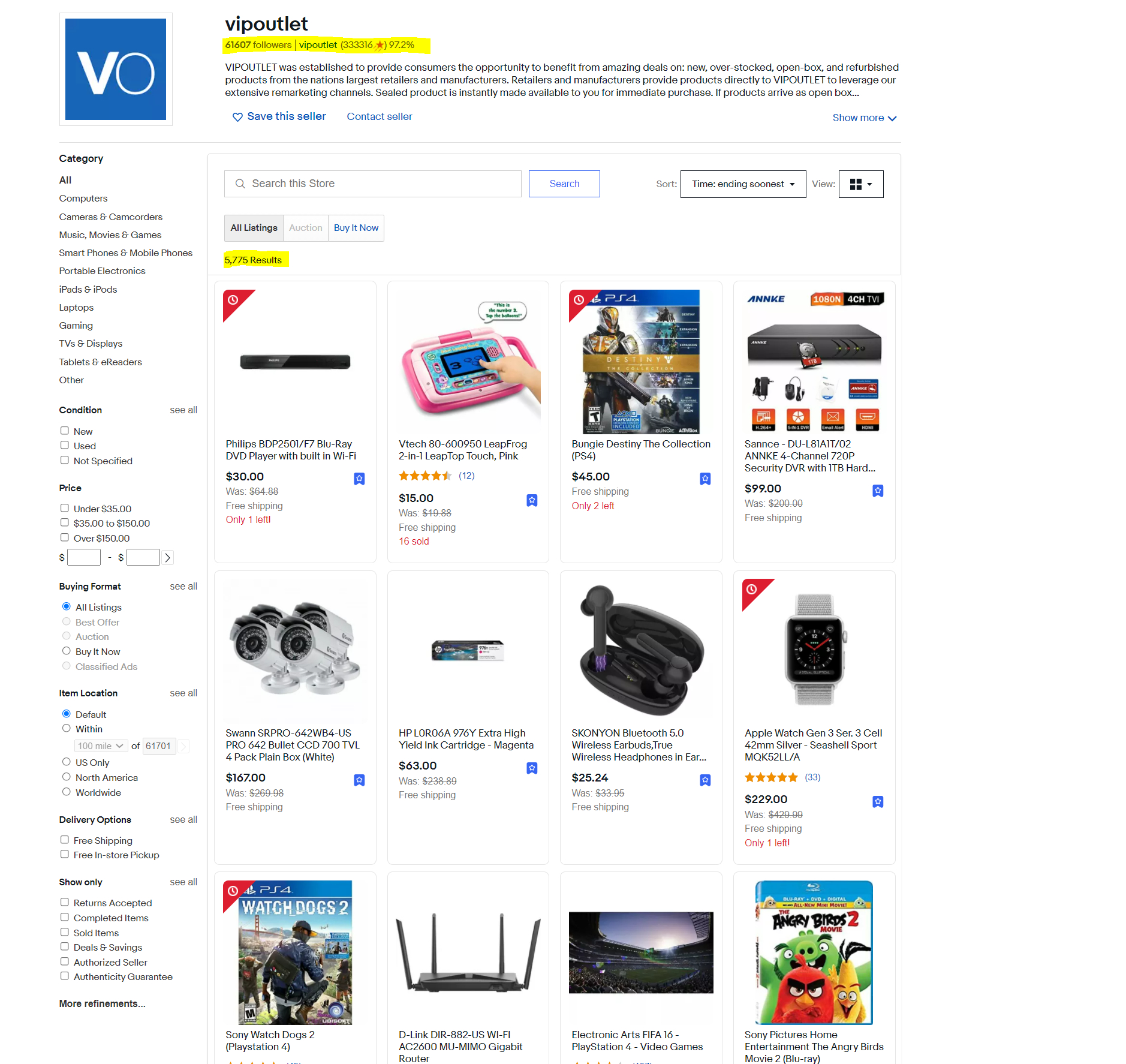Screenshot of VIP Outlet Website on a Desktop or Laptop

This image captures a screenshot of the VIP Outlet website as displayed on a desktop or laptop computer. Located in the upper left corner of the page, the VIP Outlet logo is prominently featured. The logo consists of a blue square background with the letters "V" and "O" in a white font, where the "V" is bold and the "O" is in a regular weight.

The title of the page, "VIP Outlet," is displayed in black text on a white background. Directly beneath the title, it is noted that the store has 61,607 followers. A brief description of VIP Outlet is provided, explaining that the site was established to offer consumers great deals on new, overstocked, open-box, and refurbished products from the nation's largest retailers and manufacturers. Retailers and manufacturers supply these products to VIP Outlet to take advantage of the platform's extensive remarketing channels. Sealed products become available for immediate purchase.

Below this description, there are two interactive buttons: "Save this seller" and "Contact seller." The main content of the page showcases various product images, including sound bars, DVR recording boxes, PlayStation 4 games, Blu-rays, routers, headphones, watches, ink cartridges, and various electronic devices. This diverse selection highlights the range of electronics and accessories available from VIP Outlet, inviting users to explore and take advantage of the deals offered.